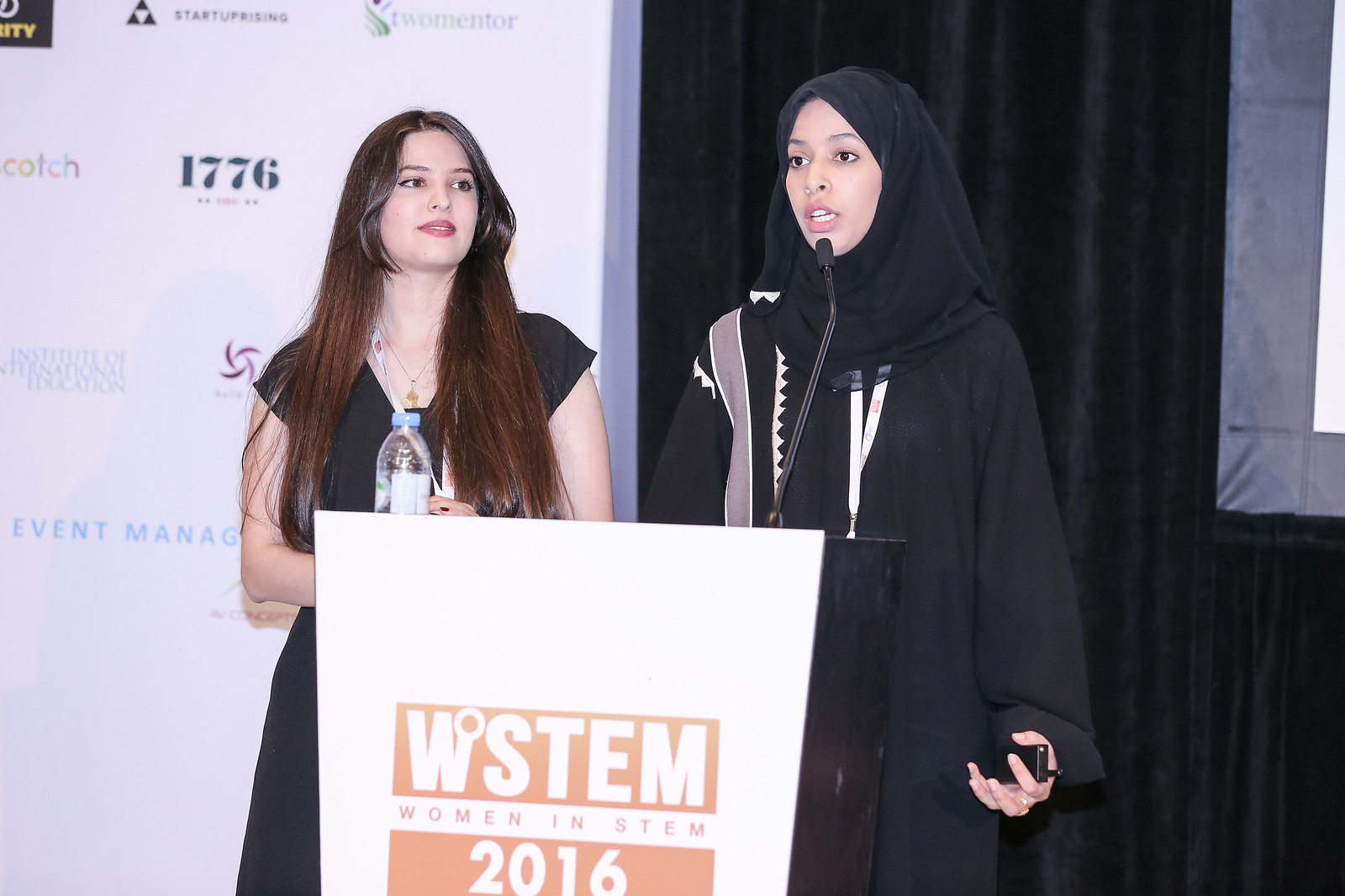The image depicts two women giving a speech behind a white podium adorned with a blue banner logo. The logo displays the white text "WSTEM," orange text "WOMENINSTEM," and the white text "2016.” The woman on the left has very long brown hair and is wearing a v-neck black dress with short sleeves. She is smiling and facing towards the right side of the picture, with a white lanyard with red font around her neck. In front of her is a water bottle. The woman on the right is wearing a black headdress, a long-sleeved black robe with a small purple stripe, and a white lanyard with orange font. She appears to be holding a PowerPoint clicker in her right hand. Behind them, a black curtain covers the stage wall. To the left side of the image, a poster displays various business logos with text including "start something," "uprising," and "1776," alongside other advertisements, though some text is partially cut off due to the angle of the photo.